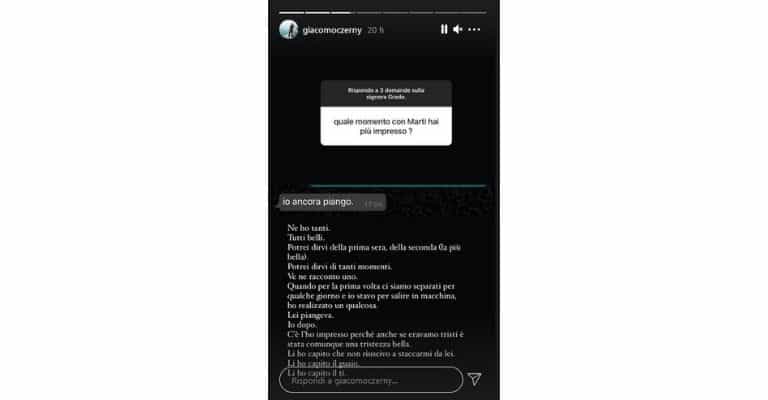This image appears to be a blurred screenshot of a computer or cell phone screen, likely from Instagram. It features a mix of text and graphical elements, predominantly in white, gray, and black colors. The image begins with a thumbnail photo in the upper left-hand corner, accompanied by white text presumably indicating the name of the user who posted. Next to the user’s name, it mentions the number '20,' possibly indicating that the post was made 20 hours ago. The navigation and notification buttons are located in the upper right-hand side.

Below the user’s information, there is a block of text or graphical elements. This block is segmented into parts with a black top and white text, followed by a white region with black text. The exact content is unclear due to blurriness and the foreign language used. There is a noticeable medium blue line spanning across the page, functioning as a separator. Below this line, there is a black title bar with white lettering, then several rows of text in varying lengths, flush left. 

The bottom section of the image contains additional elements, including more text blocks and graphical features such as an oblong circle and a small triangle. The layout follows typical Instagram formatting, with a consistent arrangement of text and a send button situated at the lower right.